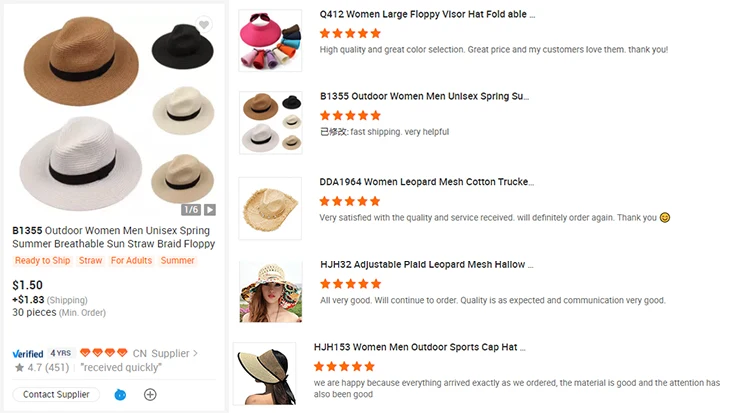This image, captured against a plain white background, is a screenshot of an online store. Prominently displayed in the upper left corner are five images featuring various outdoor hats. The first hat on the top left is brown with a blue border, followed by a dark black hat, and a cream-colored hat, among others. The accompanying product description reads, "B1355, outdoor women, men, unisex, spring, summer, breathable, sun, straw, braid, floppy." Below this description, the price is listed as $1.50, with a highlighted orange text that declares the items are "Ready to Ship." Additionally, it mentions "Straws for adults and summer." The product boasts a review rating of 4.7 out of 5 from 451 reviews. To the right side of the screenshot, more purchasing options are visible, featuring items like a "Women large floppy visor hat foldable," a "Women leopard mesh cotton trucker," and a "Women men outdoor sports cap."